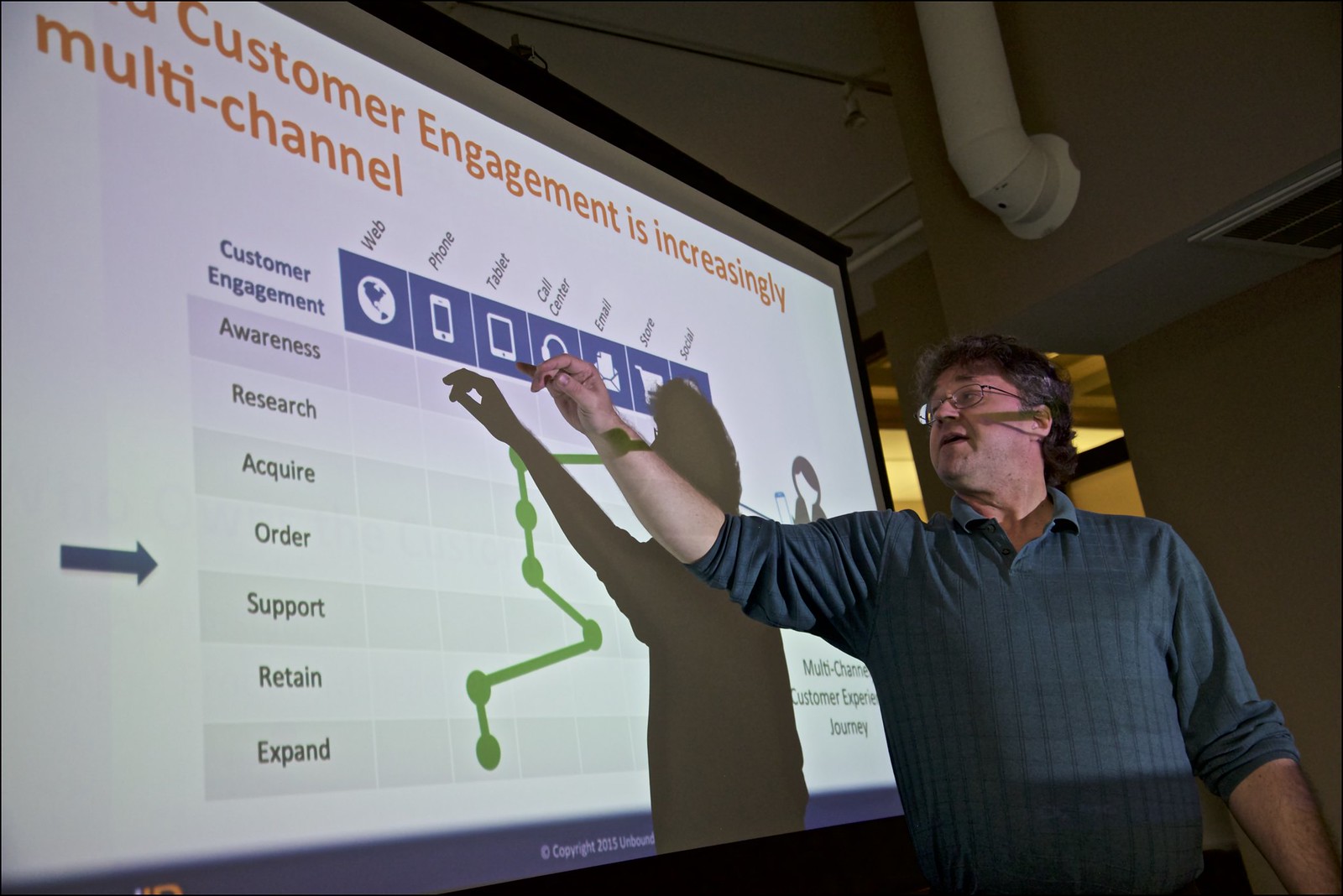In an indoor conference room, an Asian man slightly overweight, stands in front of a projector screen giving a corporate presentation. He is dressed in a dark blue, long-sleeve, collared shirt with the sleeves rolled up and black pants, and he wears glasses. A microphone is attached to him as he speaks, and he uses a pen as a stylus to point to various elements on the screen. One of his hands is raised, touching the screen where information is projected. The screen displays the phrase "Customer engagement is increasingly multi-channel" in orange over a white background. 

A detailed chart beneath this headline outlines the stages of customer engagement: awareness, research, acquire, order, support, retain, and expand. Corresponding with these stages are various channels, listed horizontally at the top of the chart: web, phone, tablet, call center, email, store, and social. Each of these channels is represented by an accompanying graphic—earth for web, phone for phone, tablet for tablet, speaker for call center, envelope for email, shopping cart for store, and another graphic for social. To the right, next to the blue tabs, is a profile graphic of a woman’s face.

The man’s shadow is cast on the projector screen as he explains the multi-channel customer experience journey, emphasizing how customer engagement spans various platforms such as phone, tablet, and email.